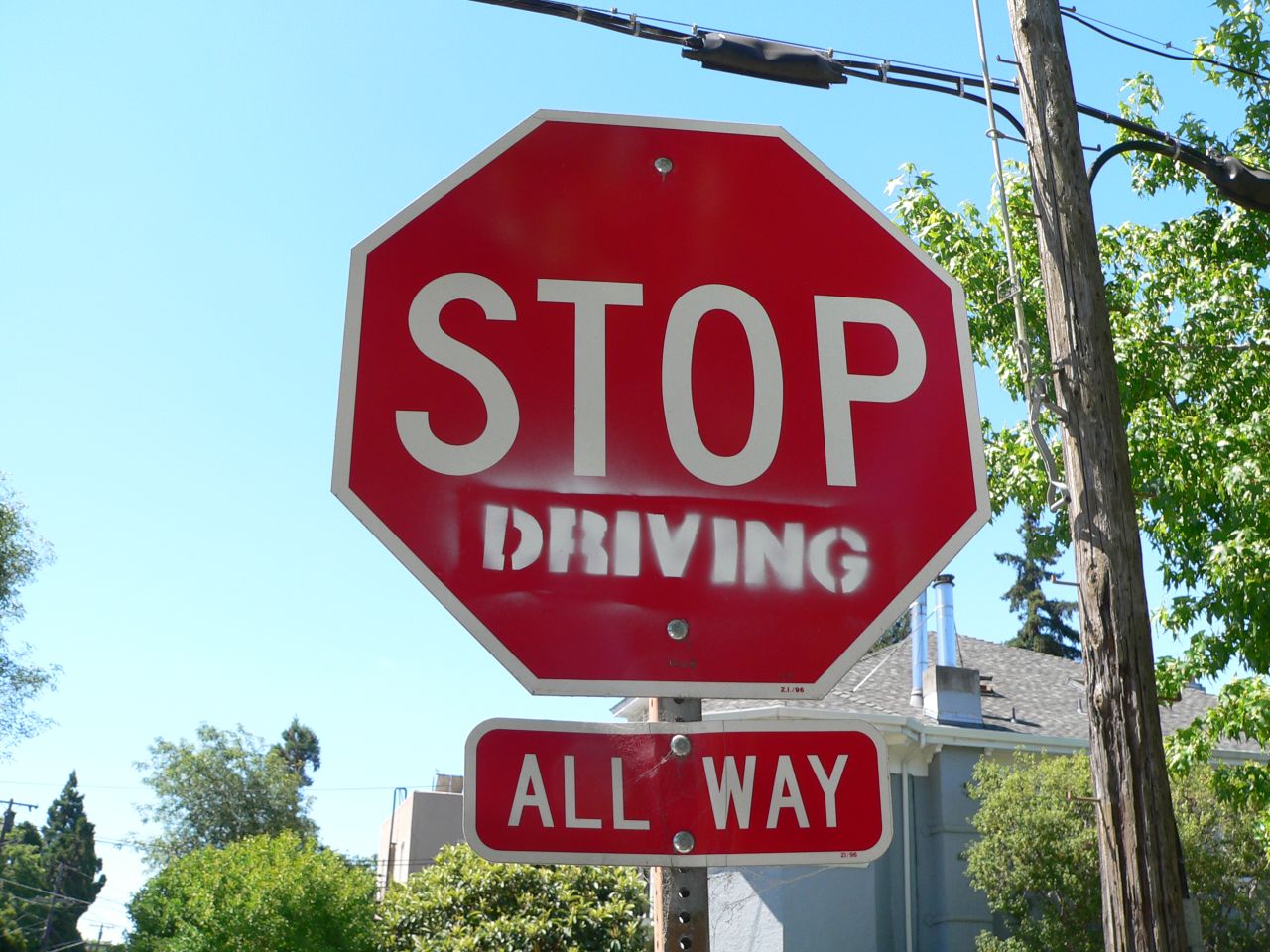This image captures a modified stop sign from a low-angle perspective against a backdrop of a clear blue sky. The standard red octagon-shaped stop sign prominently displays the white letters "STOP." Below this, the word "driving" has been added in white stenciled spray paint, transforming the message into "STOP driving." Beneath the stop sign, a smaller rectangular sign with a red background reads "all way," both signs being fastened to the same pole. To the right of the stop sign, a tall wooden telephone or electrical pole stands, with visible wires at its top. Behind the sign, you can see the blue exterior of a house with two chimneys protruding from the roof and surrounded by tall trees and bushes on either side.